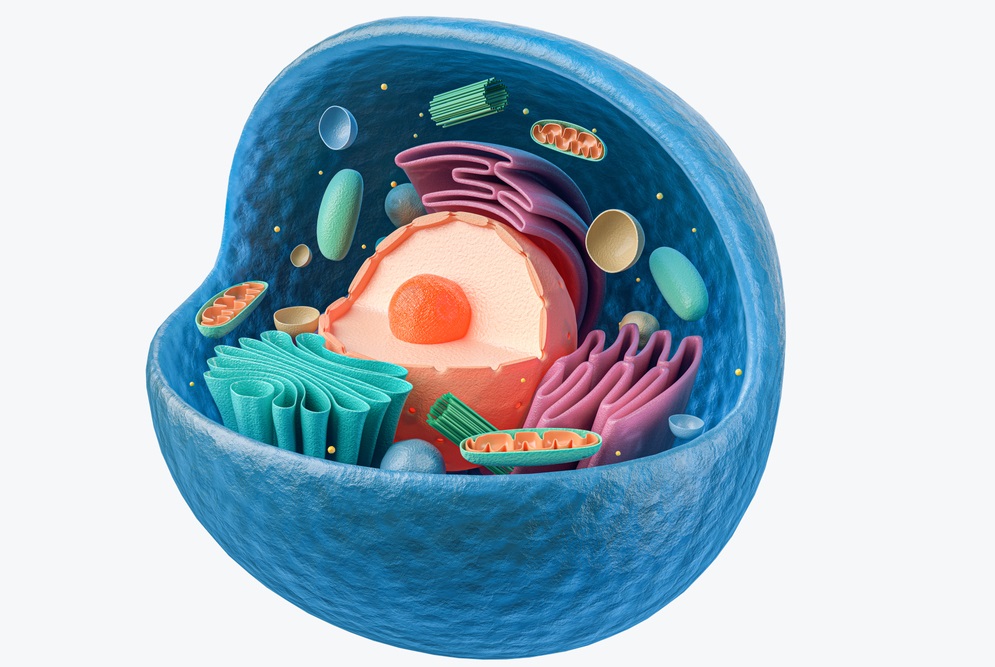The image depicts a futuristic yet slightly retro sculpture set against a completely white background. Central to the composition is an open, light blue, dimpled circular structure reminiscent of both a hollowed-out golf ball and a model of the Earth’s core. The interior of the circle hosts a miniature universe of intricate elements and vibrant colors. Dominating the center is an orange sphere within another orange ring, evoking the idea of an open egg or the Earth's core. Surrounding this core are various shapes and materials: folded structures, open elements resembling eggshells or bowls, and floating components akin to pills, pasta, and cell organelles. Colors such as teal, pink, green, cream, turquoise, purple, and blue swirl together, with notable turquoise shapes that resemble jellybeans and penne pasta, adding to the dynamic and detailed scene. The arrangement and vivid colors create an impression of suspended, detailed cellular structures, blending scientific and artistic visualization seamlessly.